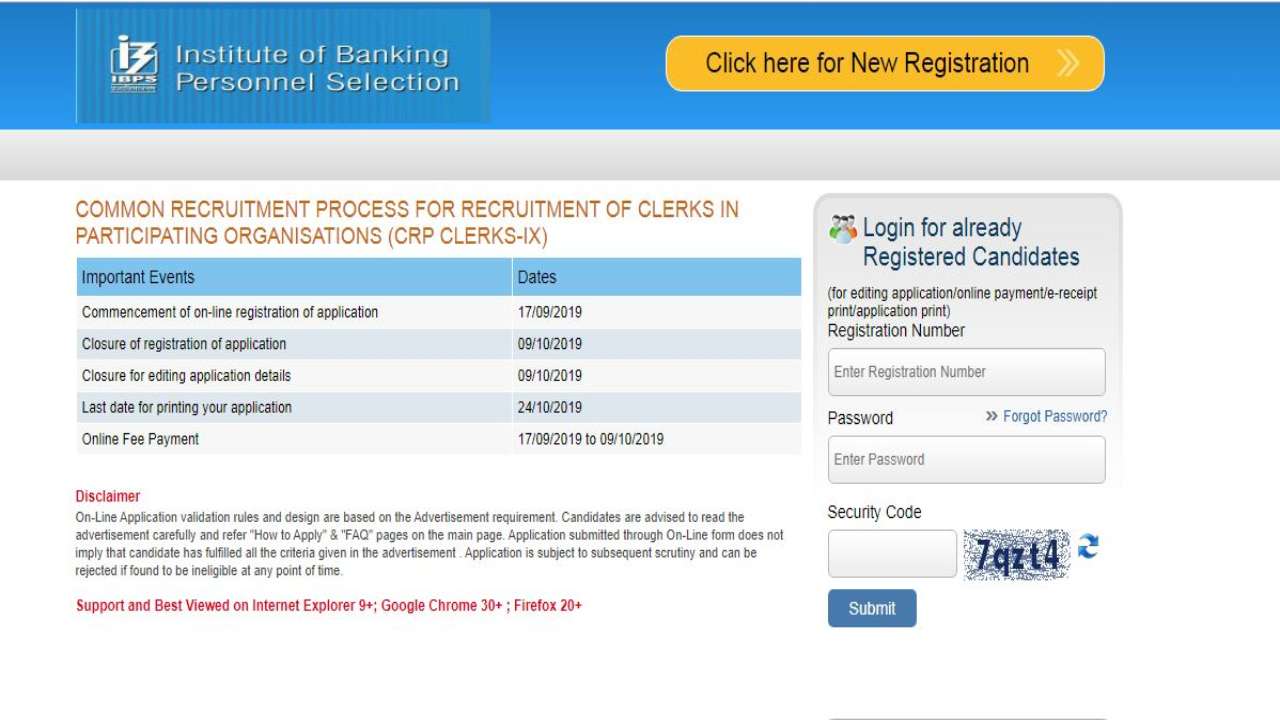The image depicts a web page from the Institute of Banking Personnel Selection (IBPS). In the top left-hand corner, within a blue, rectangular box, the institution's name is prominently displayed. This box is situated on a larger, horizontally-aligned rectangle that spans the width of the image, colored in a light royal blue. Below this header, there's a call to action in yellow text, urging users to "click here for new registration," with the clickable button also highlighted in yellow and the text in a navy blue font.

Further down, a light gray rectangular section stretches across the image, featuring the heading "Common Recruitment Process for Recruitment of Clerks in Participating Organizations," followed by "(CRP Clerks - IX)" in a brownish font. Below this section, another subsection lists "Important Events" along with corresponding dates, enumerating five specific items and their respective timelines.

In the very bottom left-hand corner, there is a disclaimer. The word "Disclaimer" is written in red, while the accompanying paragraph is in black text, providing information about optimizing viewing on Internet Explorer and Google Chrome, with emphasis text also in red.